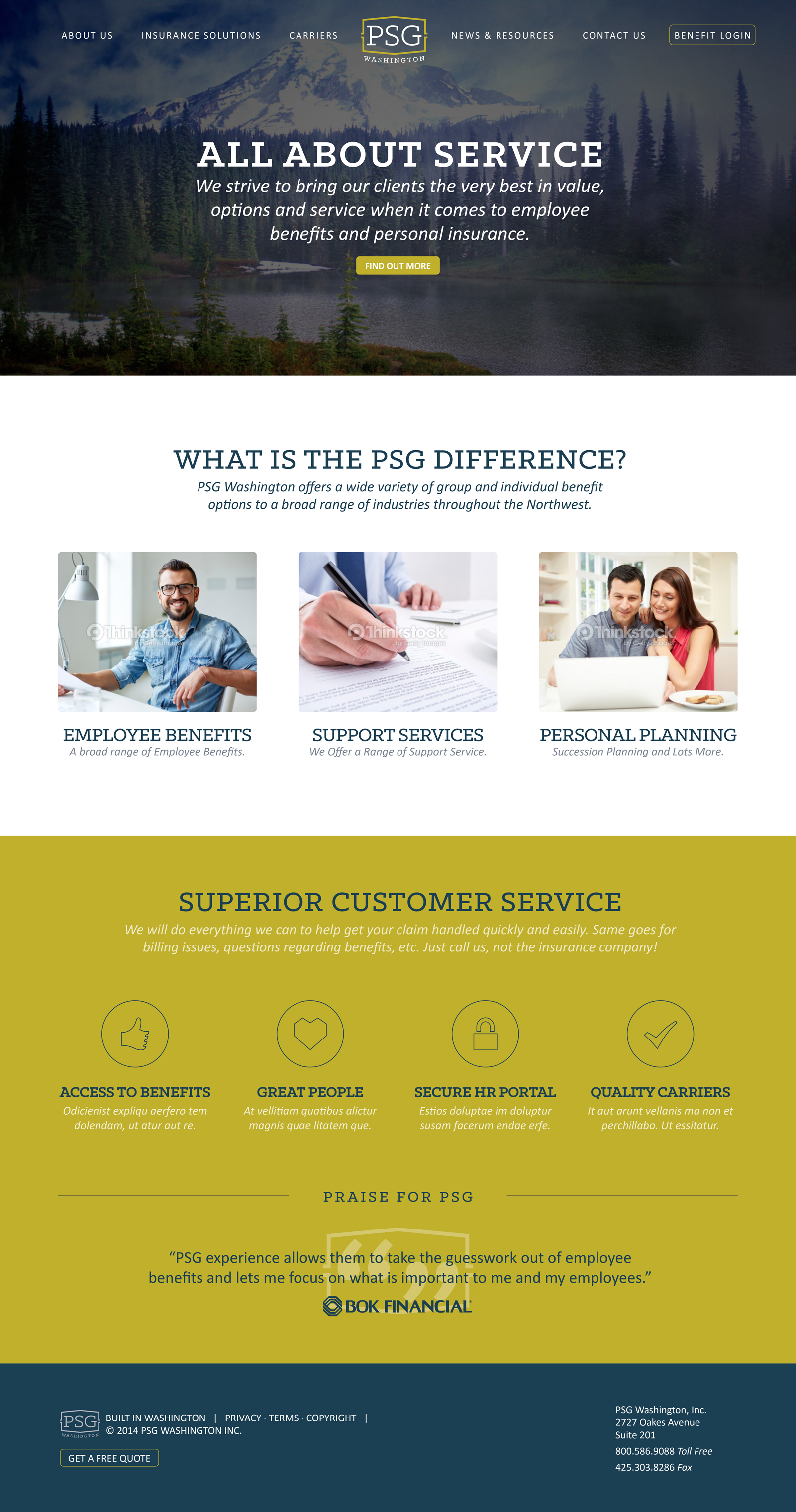Professional Service Group (PSG) Washington is dedicated to offering top-tier service solutions for all our clients. Specializing in employee benefits and personal insurance, PSG provides a wide variety of group and mutual benefit options across a broad range of industries throughout the Northwest.

[In the Image: An individual with a blue shirt, pockets, glasses, and a beard is leaning on a chair. A lamp is visible in the background, illuminating the setting which includes a mountain, trees, and water, symbolizing the serenity and scope of PSG's services.]

PSG Washington prides itself on delivering exceptional value, diverse options, and top-notch service. Our commitment shines through in our extensive support services, including personal planning, succession planning, and employee benefits management. For any billing issues, questions, or claims, our dedicated customer service team is here to assist you promptly and efficiently, ensuring you never have to deal directly with the insurance company.

We emphasize secure HR protocols and quality care, offering clients unparalleled access to benefits. The PSG difference lies in our experienced team, which is continually striving to meet and exceed the needs of our clients with great people and secure, high-quality service.

Discover more about what sets PSG Washington apart. [Highlighted by a yellow rectangle] The PSG experience allows us to extend optimal service, making your satisfaction our highest priority.